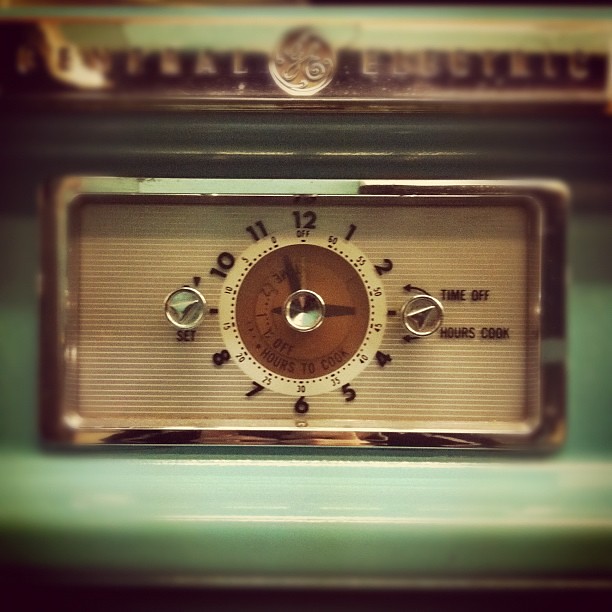This is a detailed color photograph taken indoors of a vintage clock and timer mounted on an antique General Electric stove. The clock is integrated into a green porcelain surface, and at the top of the image, the logo "General Electric" is visible in the center. The clock face is housed within a chrome-outlined rectangular box with slightly rounded corners. The clock face itself is light brown with thin white horizontal stripes. The analog clock displays traditional black numbers from 1 to 12 around its round surface, with additional timer markings in increments of 5 minutes from 60 to 0, starting clockwise from the top. The hour and minute hands are black, indicating approximately five minutes until three. Two chrome knobs, one labeled "set" and the other "time off," are positioned at the top right of the clock face, near text that also includes "hours" and "cook." The photo is slightly blurry at both the top and bottom, giving a soft focus to the green porcelain and the surrounding area.